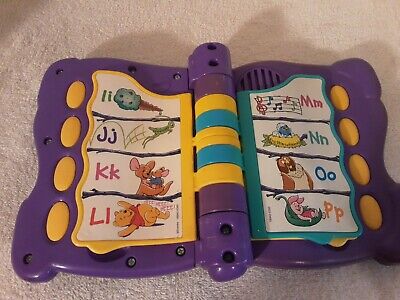The image depicts a rectangular, plastic children's toy that resembles a book and is designed to assist with learning the alphabet. The photograph, taken indoors on what appears to be a densely packed light cream or light salmon pink carpet, shows the toy fully opened. The toy prominently features a purple base with yellow and turquoise accents. On either side of the toy are four yellow, oval buttons, each correlating to a picture that teaches a different letter of the alphabet. On the left side, the letters I, J, K, and L are accompanied by images such as an ice cream cone for 'I'. On the right side, the letters M, N, O, and P are represented with corresponding pictures, including a musical note for 'M' and Piglet from Winnie the Pooh for 'P'. The colorful and engaging design is reflective of its function as a talking educational aid for young children.